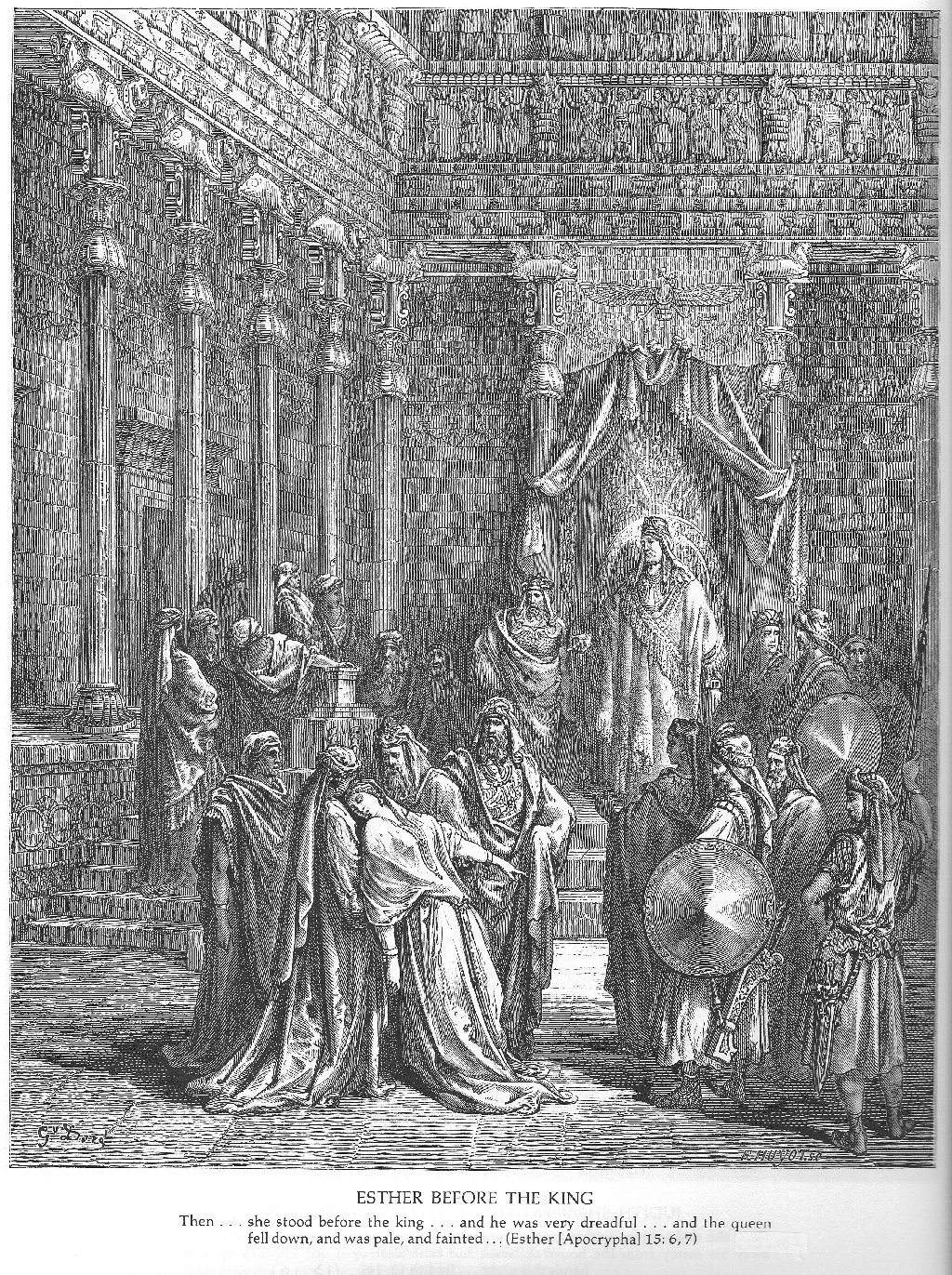This is a highly detailed black and white print, likely a pen or etched drawing, illustrating a scene from the Apocryphal book of Esther, chapter 15, verses 6 and 7. The image captures the dramatic moment described in the text. In a grand palace hall reminiscent of Roman architecture, with imposing columns and intricate stonework, a regal king stands at the top of a set of steps, under ornate curtains. He is flanked by two similarly dressed men, all wearing detailed robes and headdresses.

In the foreground, Queen Esther has fainted and is being supported by two men also donned in robes. She has long hair and her arm points downward as she swoons. To her right, a group of soldiers with visible shields, quivers, and scabbards stand in attention. Behind her to the left, additional figures—including what appear to be guards—stand near the massive columns that support the structure. The entire scene is rendered with fine, intricately drawn lines, capturing the tension and gravity of the moment as Esther appears before the dreadful king. At the bottom of the image, a white bar contains the text: "Esther before the king. Then she stood before the king and he was very dreadful, and the queen fell down and was pale and fainted."